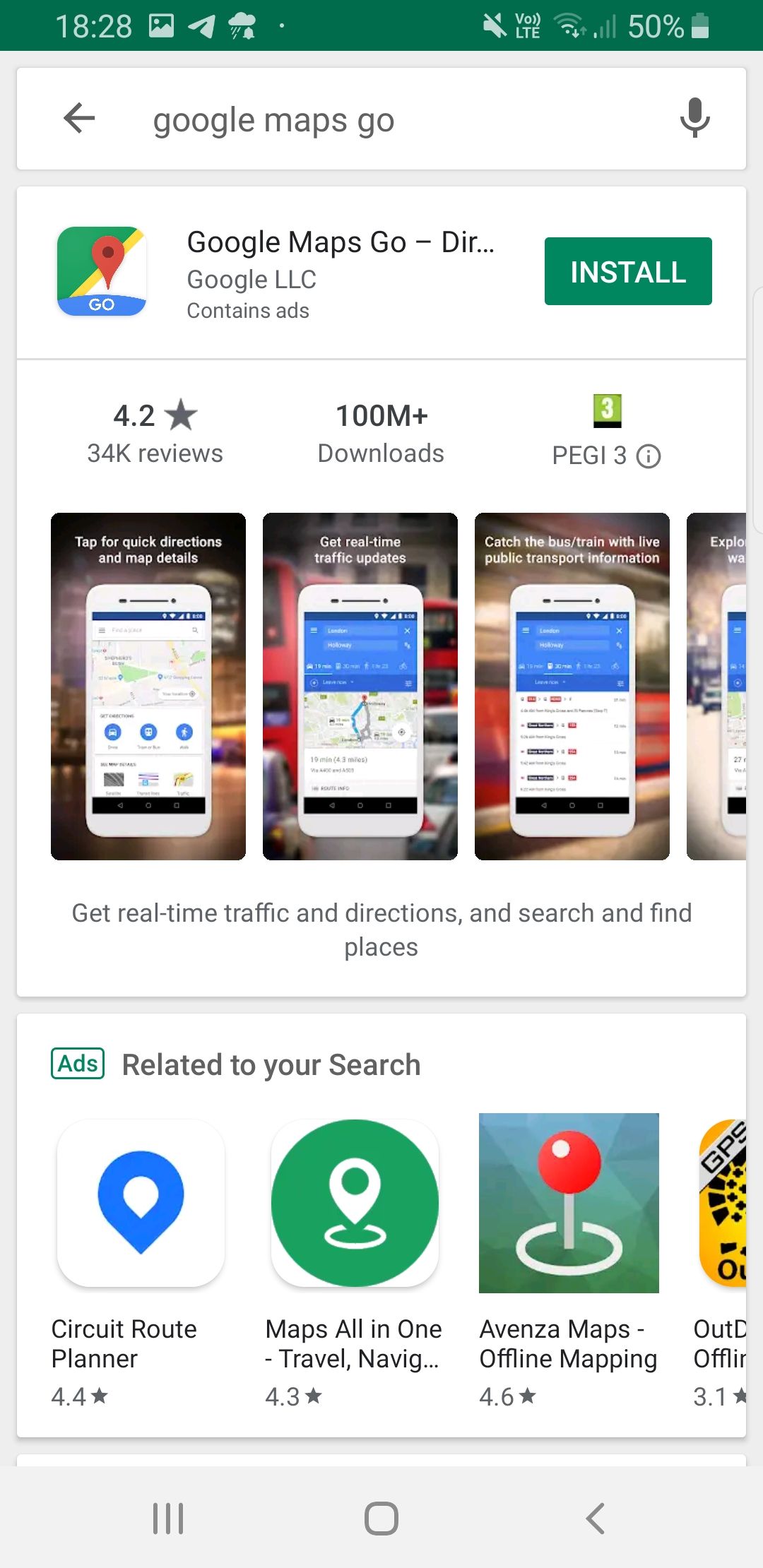In this image, we see the time displayed as 18:28 at the top, and the phone battery is at 50%. The screen shows Google Maps Go in the search bar, and the first result is the Google Maps Go app, accompanied by its icon. Below the icon, there's a green rectangular button that says "Install." The app has a rating of 4.2 stars with 34k reviews, over 100 million downloads, and is rated PEGI 3. 

The description section displays three images of an iPhone with maps on the screen, captioned with features like "Get real-time traffic and directions" and "Search and find places." Beneath this section, there is a label "Ads related to your search" showing various app suggestions against a white background. These include Circuit Route Planner, featuring a blue location icon, Maps All-In-One, with a green circle enclosing a location icon, and Events and Maps, which has a red pin needle icon.